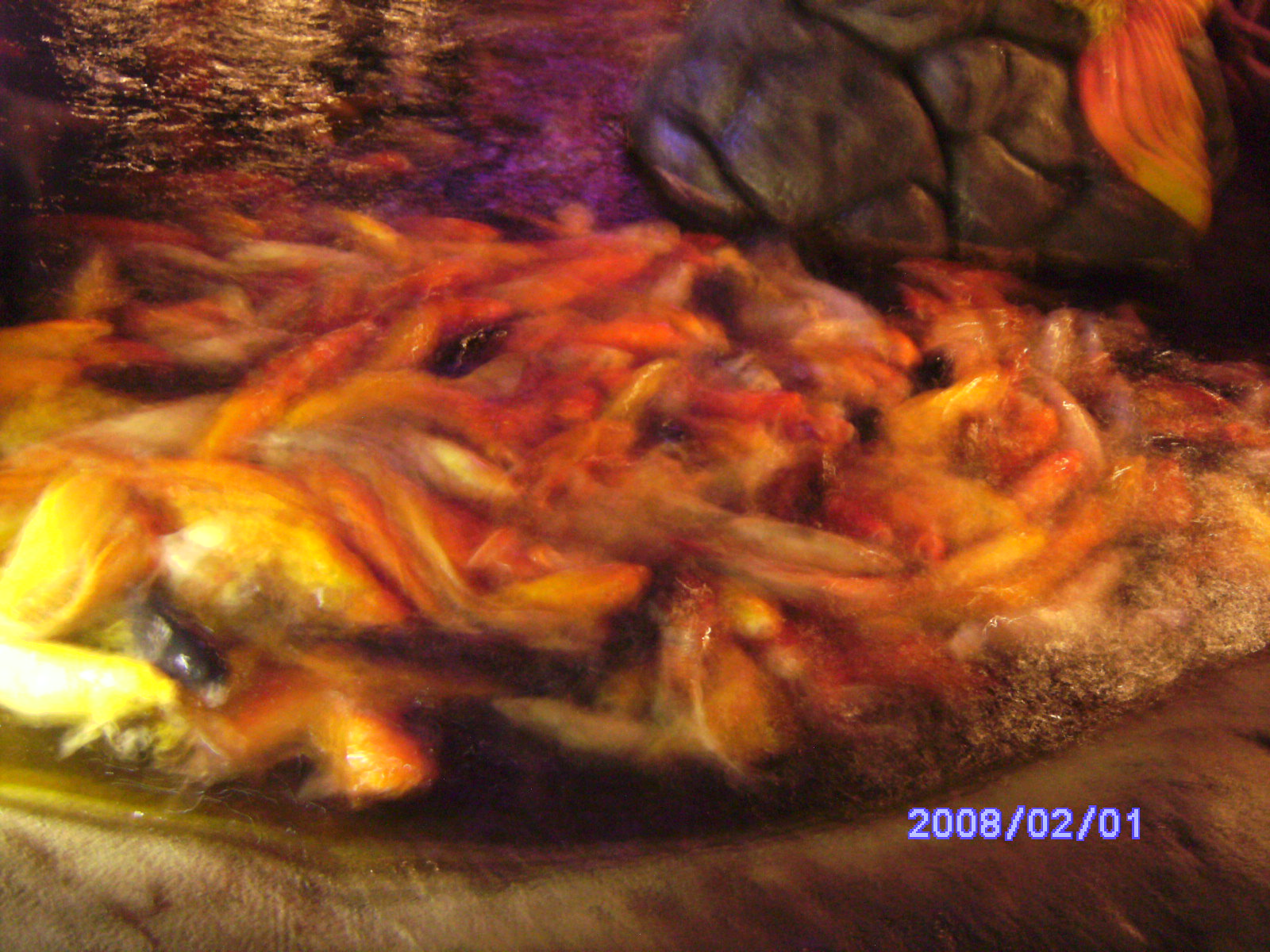The image, dated February 1, 2008 and stamped in light blue text in the bottom right corner, is notably blurry and out of focus, making identification challenging. It seems to depict an underwater scene. In the lower section of the photo, there are brownish-gray, rock-like formations with visible cracks, reminiscent of polished underwater stones. The central area features a tangled mass that appears to be a mix of twisted orange and cream-colored tentacles or worms, resembling a plate of spaghetti. To the upper right, there is a vibrant, fish-like shape with yellow, red, and orange hues, possibly resembling a fish tail or mermaid’s tail, creating an impression of motion as if swimming upwards. The backdrop includes a wave-like water texture in shades of purple and dark gray, contributing to the overall impression of an underwater environment. The visual chaos is accentuated by varied textures and colors, ranging from yarn-like strands to the illusion of brain matter, stitching together an intricate and perplexing underwater vista.